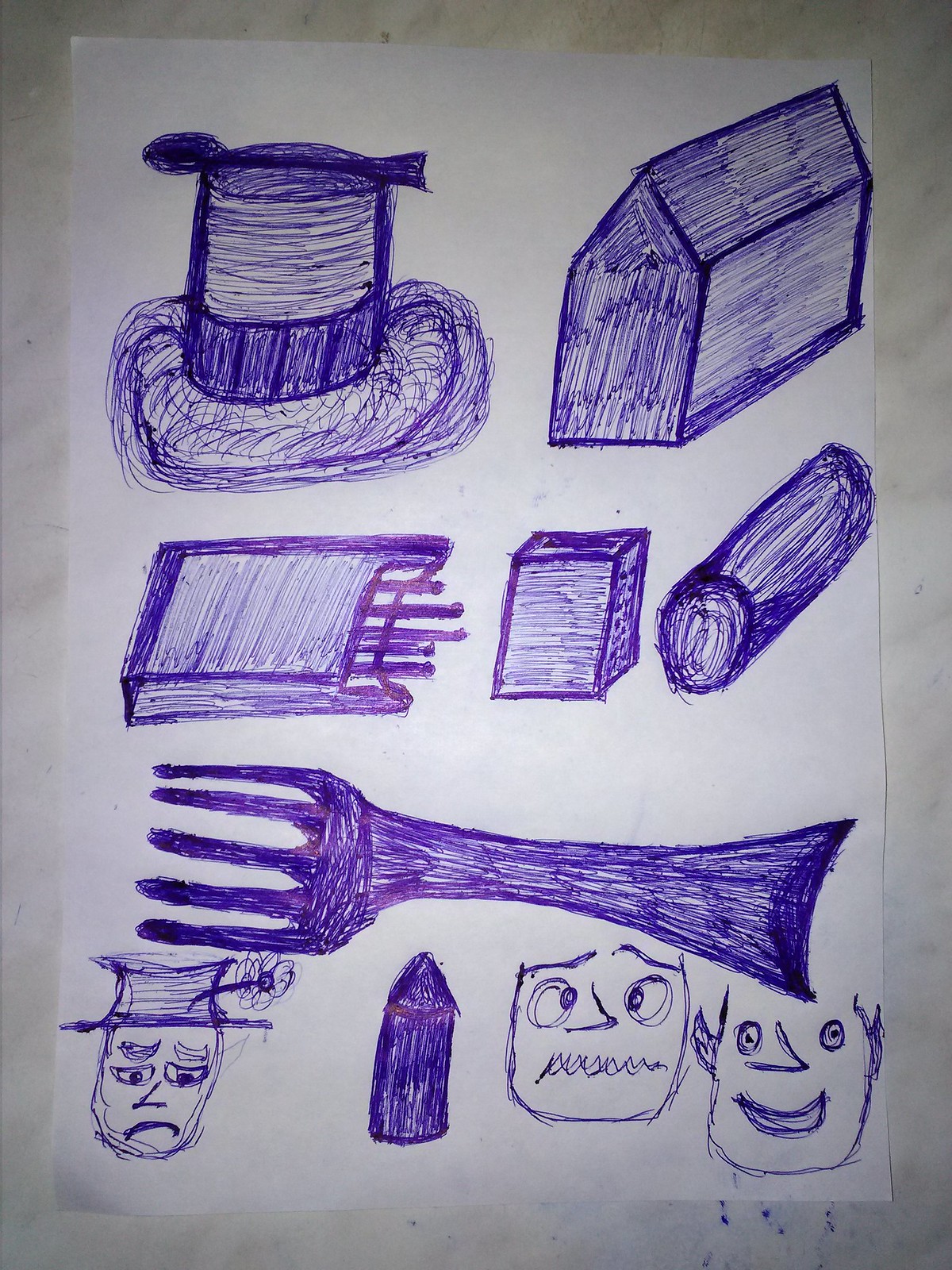This photograph captures a white piece of paper, laid flat on a gray background, adorned with various blue ink drawings. At the top left, there is a detailed sketch of a top hat with a distinctive band, curiously balanced with a spoon on the top. Adjacent to it sits a tall structure resembling a barn. Below these, a matchbox or cigarette box emits lines suggestive of contents within, followed by another small square box and a cylindrical object. Dominating the center of the page is a wide pitchfork with five tines, artistically extending across the horizontal width of the paper. At the bottom, a series of three roughly sketched faces reveals quirky, expressive features: one wears a hat adorned with a flower and frowns, another appears to have a mouth zipped shut, and the last one smiles. Additionally, there's an enigmatic drawing of what resembles a bullet. These spontaneous, passionate doodles, likely from a non-expert yet enthusiastic artist, offer an intriguing peek into the whimsical and varied sketches created in a moment of free expression.